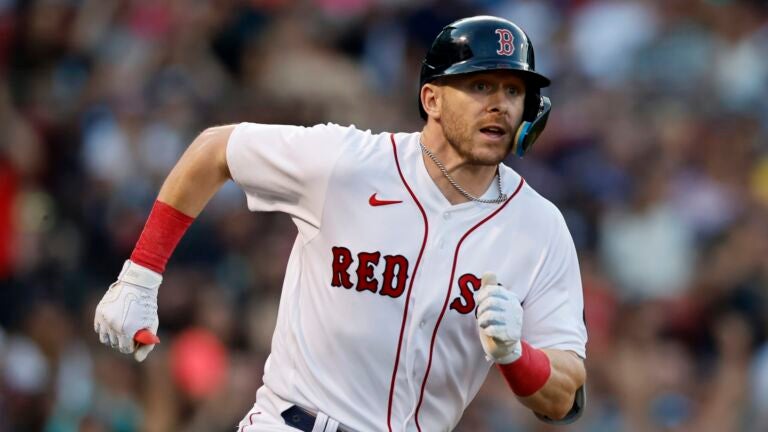This photograph showcases a Caucasian Red Sox baseball player mid-game. He's captured in motion, wearing a pristine white Red Sox uniform with red trim and the team's name emblazoned in red across his chest. The uniform features a red Nike swoosh on his right shoulder. The player’s attire is accentuated by red tape wrapped around his wrists and white gloves on his hands. In his right hand, he holds something red and pointy protruding about an inch, possibly the tip of a carrot. On his head, he dons a black helmet marked with a red "B" outlined in white, typical of the team’s gear. Around his neck hangs a silver chain, adding a touch of personal flair. The background consists of an out-of-focus crowd, blending together in a blur, placing full emphasis on the player's dynamic presence at the center of the image.